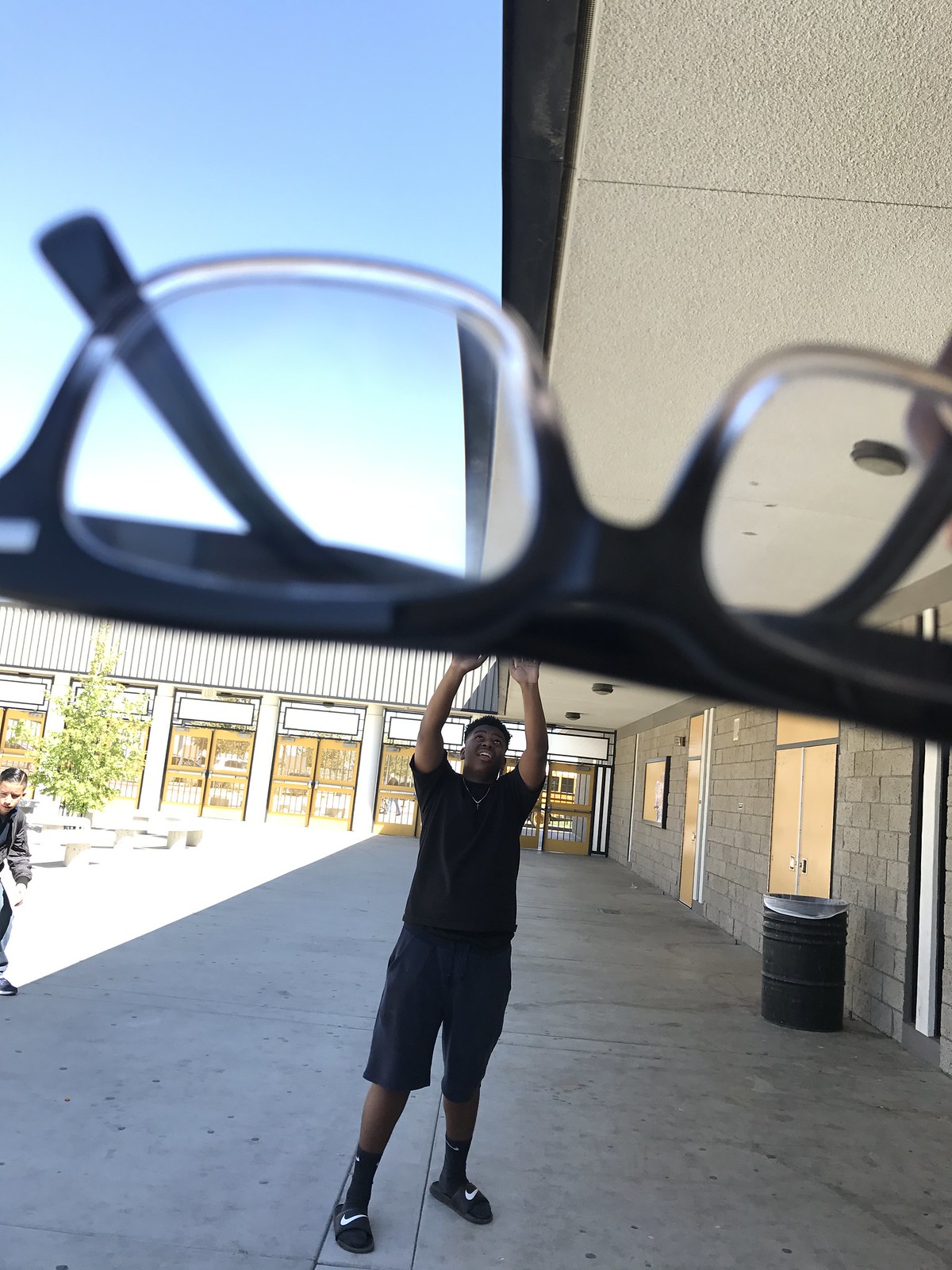This photograph captures an intriguing scene set in an outdoor plaza, likely near a school or public building. In the foreground, a pair of black-rimmed reading glasses are prominently held upside-down, creating an illusion that they obscure and interact with the background. A young African American man stands several feet away, aligned perfectly so that he appears to be holding up the glasses. He is dressed in a black short-sleeve t-shirt, blue shorts, black socks, and Nike slip-on slippers, with a gold chain around his neck. His arms are raised above his head, enhancing the playful illusion. To the right, a black trash can is positioned against a light brown brick wall with lighter brown doors. The left side of the photograph reveals a partial view of another young boy, possibly of Mexican descent. The background features a row of doors and a single green tree amidst some stone benches, with clear skies overhead, further setting the scene in a calm, open concrete plaza.